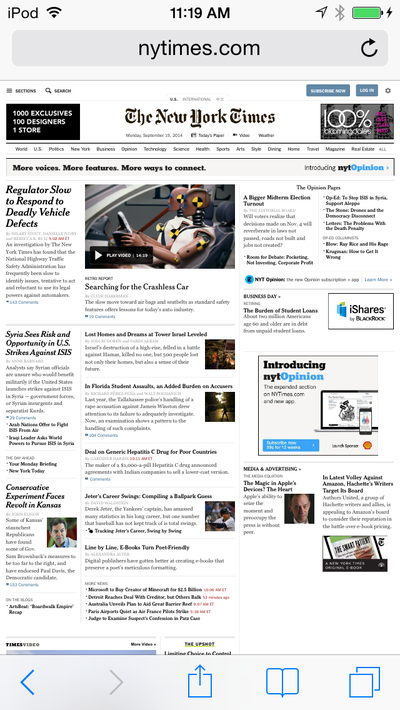This is a detailed screenshot from an iPod. At the top of the screen, the status bar shows the text "iPod," three Wi-Fi signal bars, the time "11:19 AM," a grayed-out Bluetooth logo, a directional icon, a full battery indicator with a green fill, and a lightning bolt signaling charging. Below the status bar, the web page visited is nytimes.com, identifiable by the New York Times logo in Old English text and a refresh icon to the right.

The website's main headline is prominently displayed, with advertisements bordering it: to the left, one reads "1,000 exclusive, 100 designers, 1 store," and to the right, "100% Bloomingdale's."

The navigation menu beneath the header lists various sections, including World, U.S., Politics, New York, Business, Opinion, Technology, Science, Health, Sports, Arts, Style, Dining, Home, Travel, Magazine, Real Estate, and Hall.

The web page layout mimics a traditional newspaper with a four-column design. The primary headline reads, "Regulators Slow to Respond to Deadly Vehicle Defects," accompanied by an image of crash test dummies and a playable video thumbnail. Other headlines in smaller text, such as "Syria Seeks Risk and Opportunity in U.S. Strikes Against ISIS," "Conservative Experiment Faces Revolt in Kansas," and various stories about a baseball player and other topics, populate the columns below.

The site also contains opinion pieces interspersed with ads and headlines. The bottom of the screenshot displays typical navigation icons for forwarding, backward, sharing, and copying.